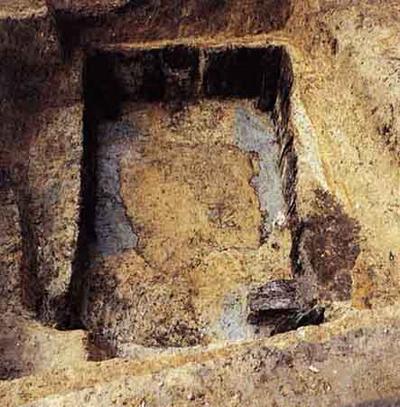This image depicts an overhead view of an ancient, gritty, stone masonry scene embedded in a dark brown wall. The central focus is a dark stone recess with an overhanging upper section, creating a shaded and mysterious cavity. Adjacent to the recess, broken stone pillars suggest a ruinous past. The outer section reveals weathered and textured stone, with shades of brown and tan adorned with scratches and indentations. The innermost section of the recess is darker, accentuated by a broken, irregular circle on its floor, hinting at its antiquity and lack of a discernible purpose. The foreground features an outcropping, potentially stairs, adding depth and architectural interest to the image. Overall, the photograph captures a rugged and intriguing historical site.